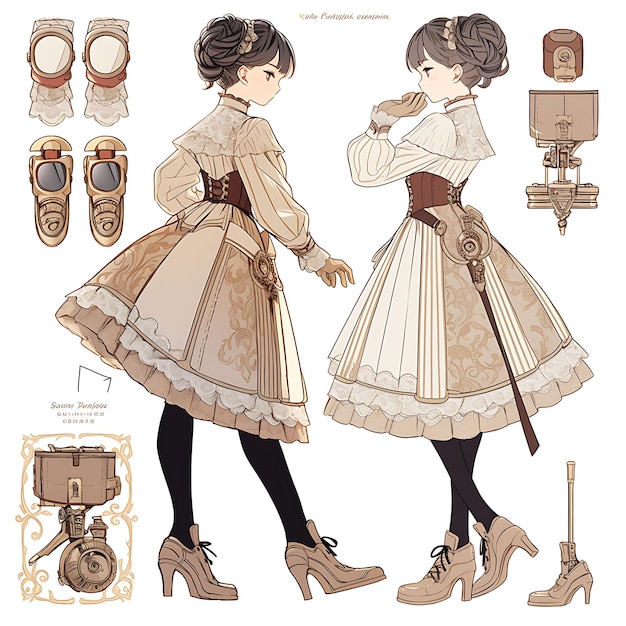The sepia-toned drawing depicts two young girls adorned in vintage, steampunk-inspired attire. Both girls, with their hair elegantly pinned up, are captured mid-interaction; each is wearing a frilly dress that falls just below the knees, complemented by puffy sleeves and tight brown cummerbunds cinching their waists. Their footwear consists of high-heeled, lace-up ankle boots, paired with black tights. The dresses feature pinstriped patterns in subtle shades of tan, transitioning from lighter to darker hues. Scattered around the central figures are magnified illustrations of various accessories they are wearing, including intricate earrings, clasps, and an odd shoe image featuring what looks like a toilet brush or a metal bar, suggesting the presence of a mechanical or robotic element to the girls. This adds a whimsical steampunk vibe to the entire composition.